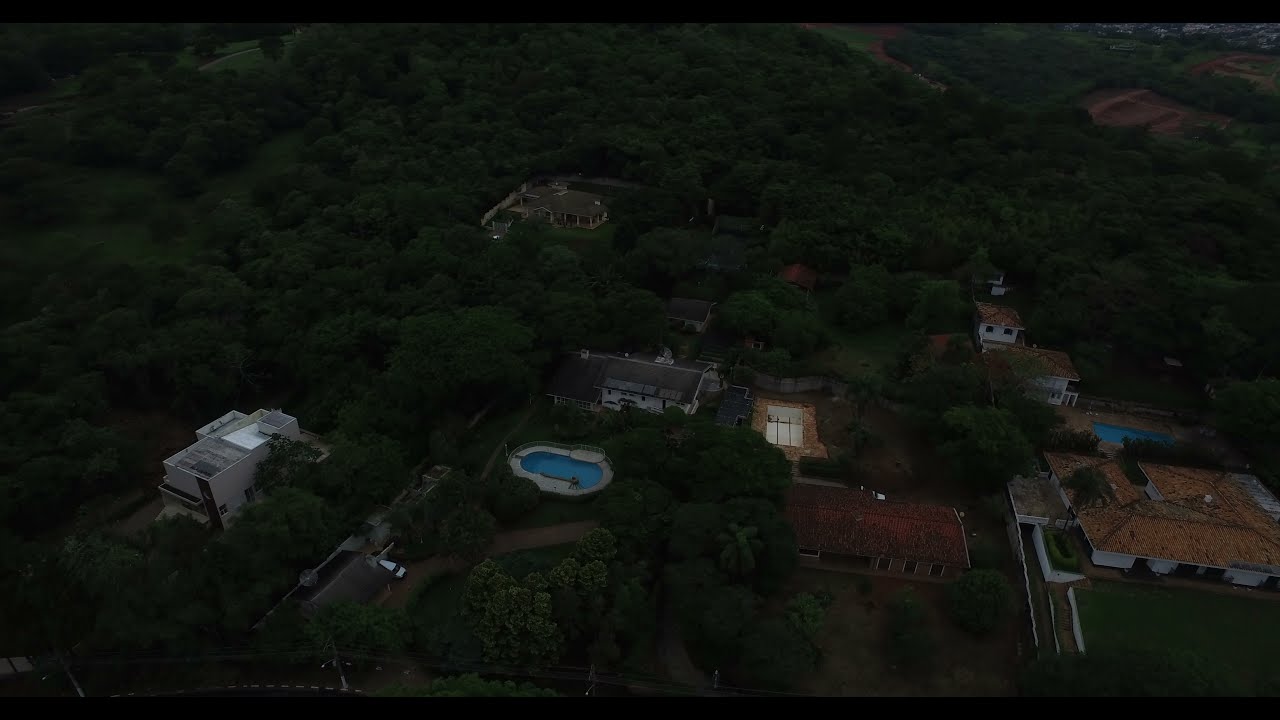This aerial color photograph, taken at night, captures a lush green landscape dotted with multiple structures, predominantly large homes interspersed among dark green trees. The image is dark, suggesting dusk or nighttime lighting conditions which obscure some details. The homes feature a mix of gray, brick-colored, and red tile roofs. Prominently, two swimming pools are visible, one near the center and another to the right, with blue water standing out against the darker surroundings. Toward the center, there appears to be a building that might be a clubhouse, flanked by a large pool and a lit tennis court. On the left side of the image, there is a white building with a possible car parked nearby, while on the right, some rooftops stand out with their brown coloration. The entire area is heavily surrounded by trees and grass, giving a sense of an opulent, tree-covered neighborhood.